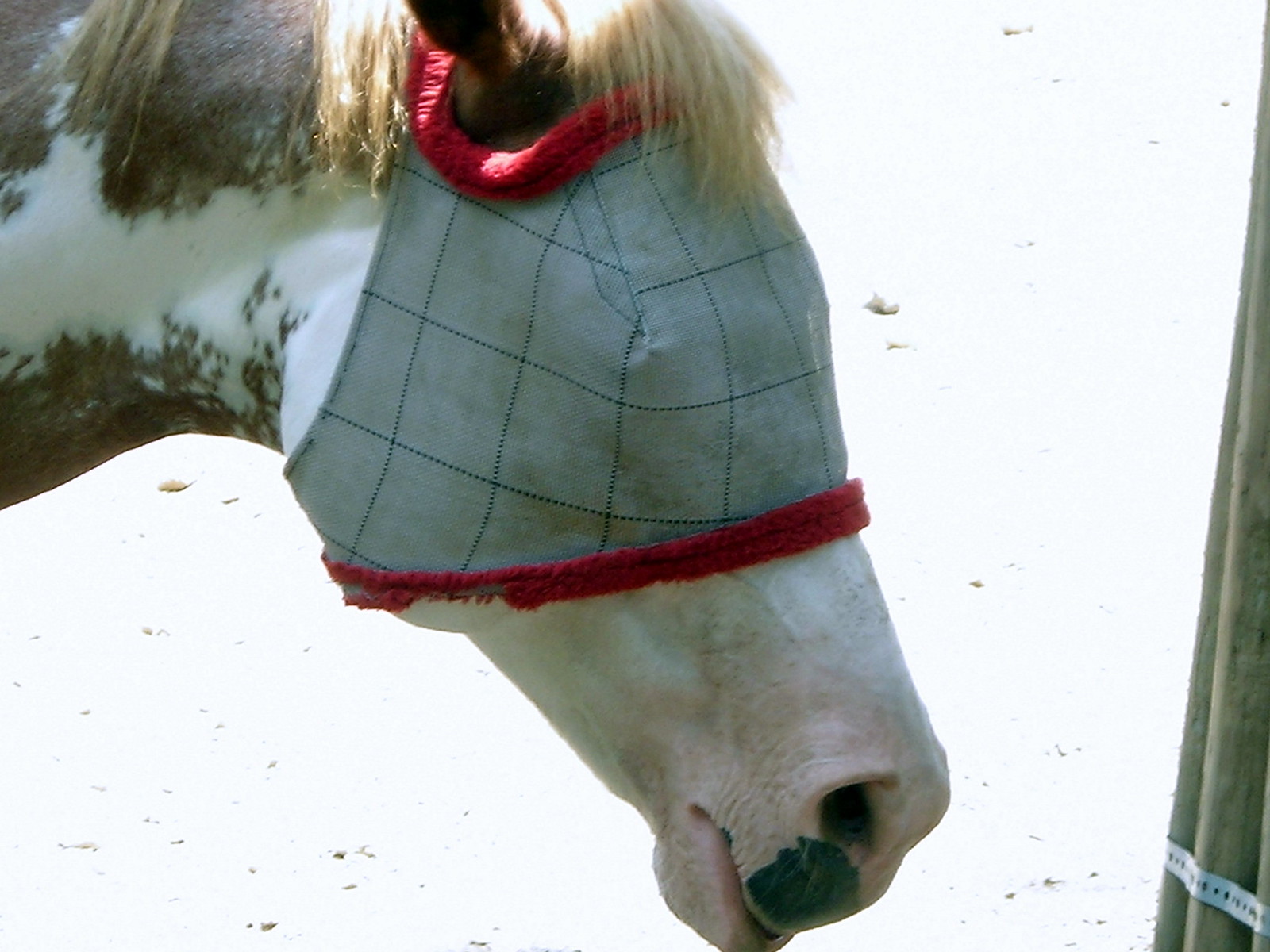In this photo, a horse's head is prominently featured against a washed-out, white background, likely due to intense sunlight. The horse has a long mane that catches the light, adding a soft glow. Its face is predominantly white with brown markings near the nose. The horse is wearing an eye mask, possibly to help mitigate anxiety or protect against the sun. This mask covers its eyes and secures around its ears, leaving the nose and mouth exposed. The mask is made of a robust, white fabric patterned with blue lines forming squares. The edges of the mask are trimmed with a soft, shaggy red material, and green stitches are visible, adding to its distinct appearance. The backdrop of the photo is extremely bright, suggesting a sunlit outdoor setting.